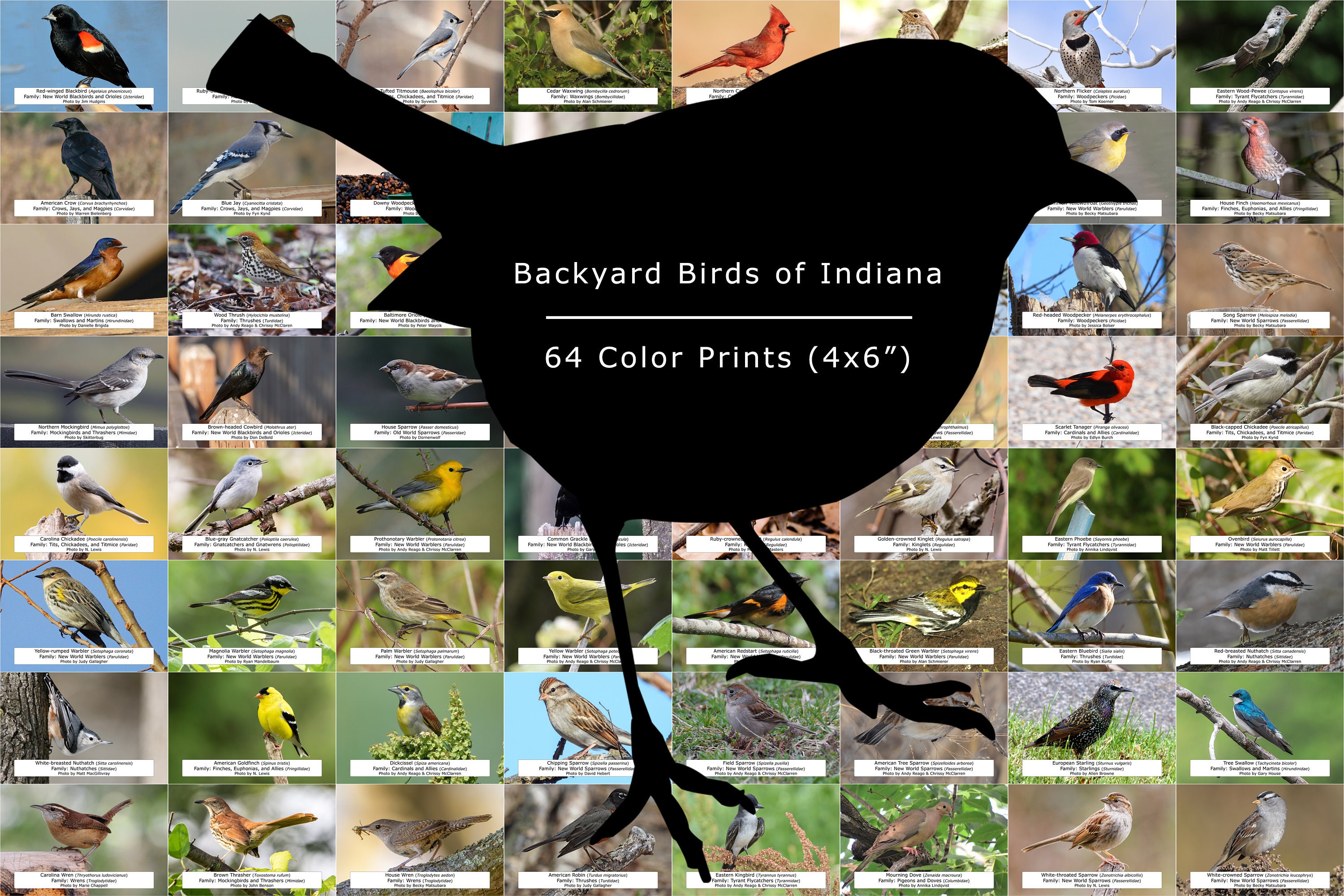This image is a vibrant rectangular collage titled "Backyard Birds of Indiana," featuring 64 color prints. The collage consists of an 8x8 grid of photographs, each depicting a different bird commonly found in Indiana. Each photo is bordered in white and accompanied by black and white text labels that provide information about the birds. The center of the collage is dominated by a black silhouette of a bird, overlaying the grid. Within this silhouette, white text reads "Backyard Birds of Indiana," followed by "64 color prints (4 by 6 inches)." The collection includes a variety of birds such as red-winged blackbirds, cardinals, goldfinches, eastern bluebirds, sparrows, and possibly flycatchers, mostly representing songbirds. The layout, vibrant colors, and detailed labeling create an informative and visually appealing presentation of Indiana's backyard bird species.